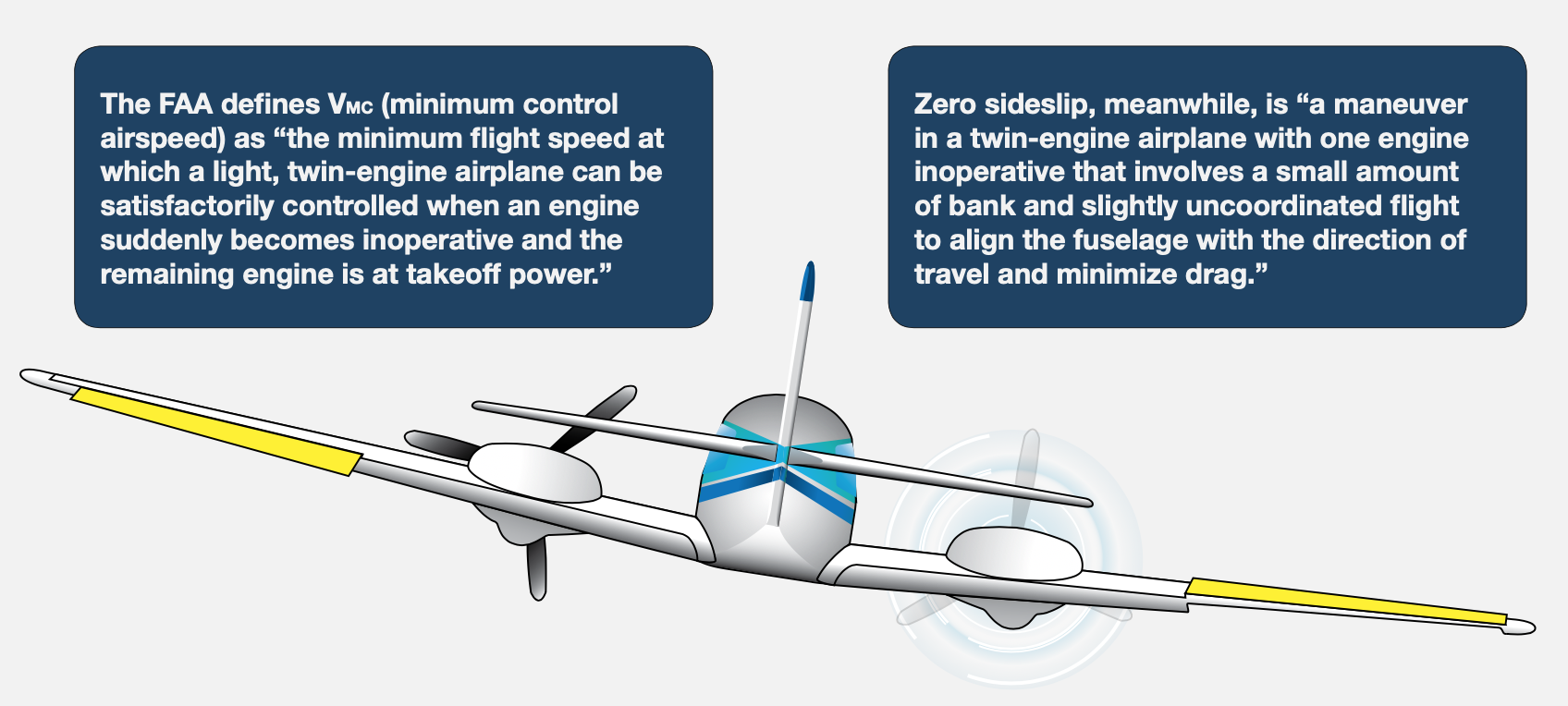The image displays a computer-generated diagram with textual information and a visual representation of an airplane. At the bottom of the diagram, there is an illustration of a grey-colored airplane viewed from the back. The airplane features yellow flaps on its wings and blue patterns on its fuselage. The background of this section is light grey. At the top of the image are two blue, rounded rectangles containing text.

The left rectangle contains the following text: "The FAA defines VMC, minimum control airspeed, as the minimum flight speed at which a light twin-engine aeroplane can be satisfactorily controlled when an engine suddenly becomes inoperative and the remaining engine is at take-off power."

The right rectangle contains the following text: "Zero side-slip, meanwhile, is a manoeuvre in a twin-engine aeroplane with one engine inoperative that involves a small amount of bank and slightly uncoordinated flight to align the fuselage with the direction of travel and minimize drag."

The diagram aims to explain key aerodynamic concepts related to twin-engine airplanes, focusing on VMC and zero side-slip conditions.